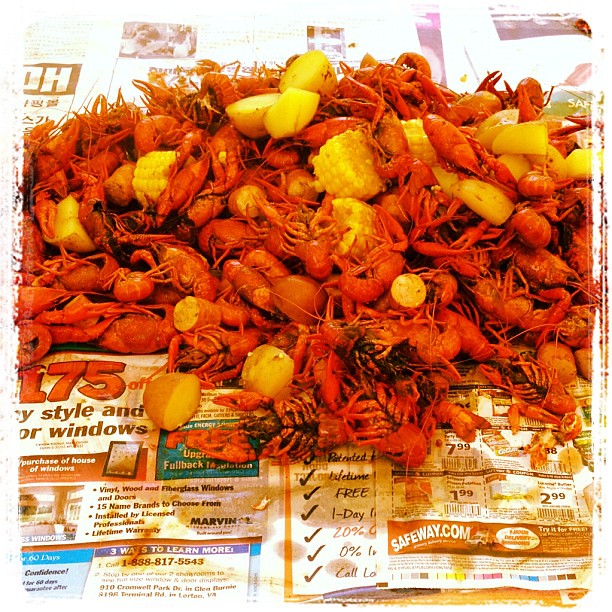The photograph depicts a vibrant and somewhat washed-out top-down view of a seafood spread, laid out on a surface covered in old newspapers. Dominating the scene is a large pile of bright red-orange cooked crawfish, their bodies curled up with visible legs and long antennae. Interspersed among the crawfish are halved potatoes and small slices of corn on the cob, adding bursts of yellow to the predominantly red-orange palette. The image appears to have an orange tinge, possibly due to the lighting, while the top section seems almost whitewashed, giving it a bright, slightly overexposed look. The newspapers underneath serve as a casual, rustic table covering for what seems to be a traditional seafood boil setup.